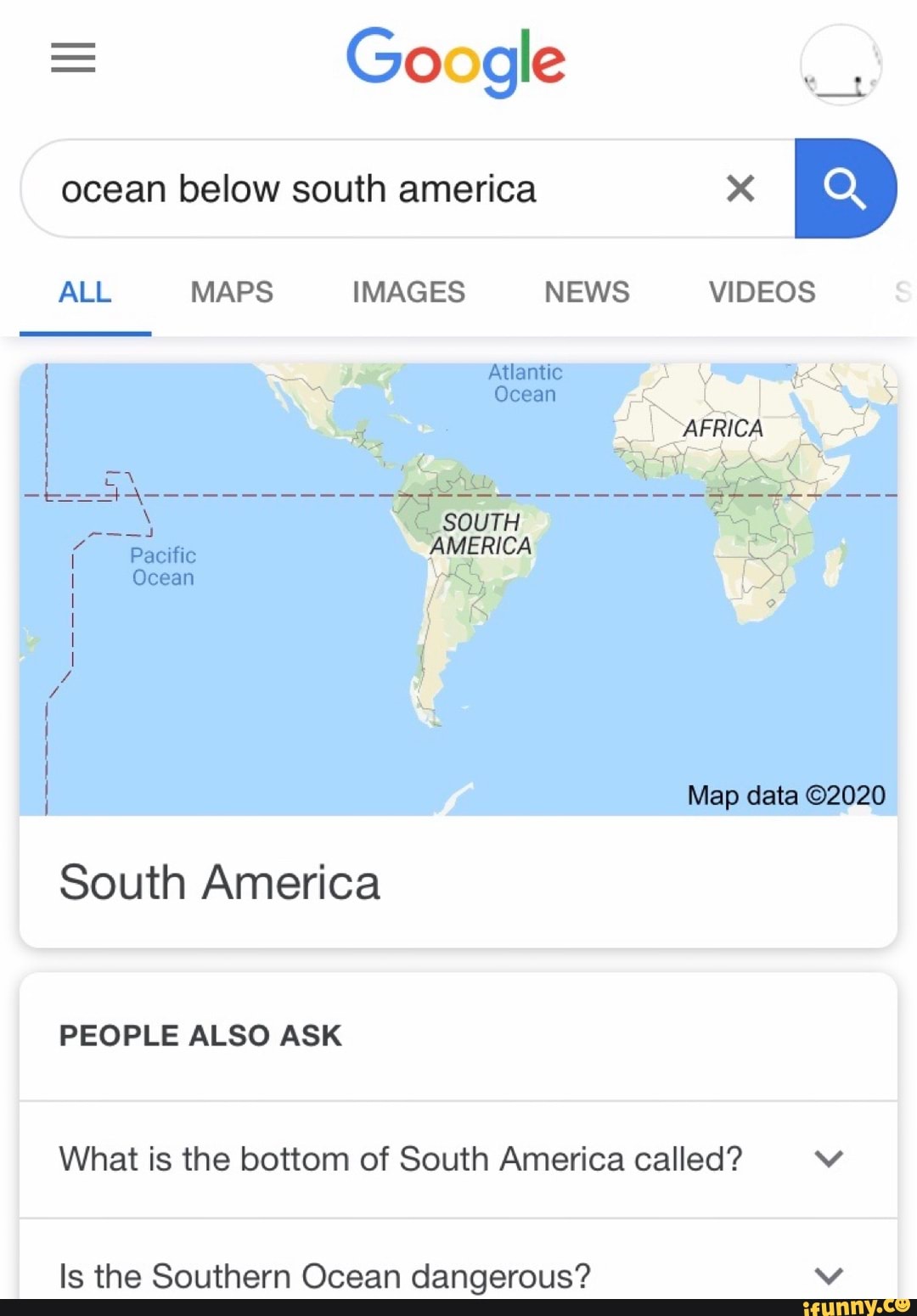The image portrays a Google search results page with a dominant focus on geographical information about South America. At the top center of the page, the familiar Google logo is displayed, accompanied by a navigation bar to its right. This bar includes a circle with an indistinguishable image inside it, commonly an account or app icon.

Directly below the logo lies the search bar, which has "ocean below South America" typed into it. Adjacent to the search bar on the right, there is a blue button with a white magnifying glass icon, signifying the search functionality.

Further down the page, several tabs are presented, offering different categories of search results: All, Maps, Images, News, and Videos. Following these tabs, a large map is displayed prominently. This map shows the equator line and prominently highlights South America, detailing the surrounding ocean. The equator cuts through the continent, visually emphasizing its geographical position.

Beneath the map lies a labeled box that reads "South America." Adjacent to this is another section labelled "People also ask," featuring dropdown menus with frequently asked questions about South America. An example of these questions includes inquiries like "What is South America?", "Where is the southernmost point of South America?", and curious questions about the dangers of the Southern Ocean.

At the bottom of the page, a black bar spans the width of the screen. In the bottom right-hand corner of this bar, the text "iFunny.co" is visible, with the 'O' stylized as a smiley face. The map itself is noted to have a copyright mark reading "map data © 2020." The general background of the page is predominantly white.